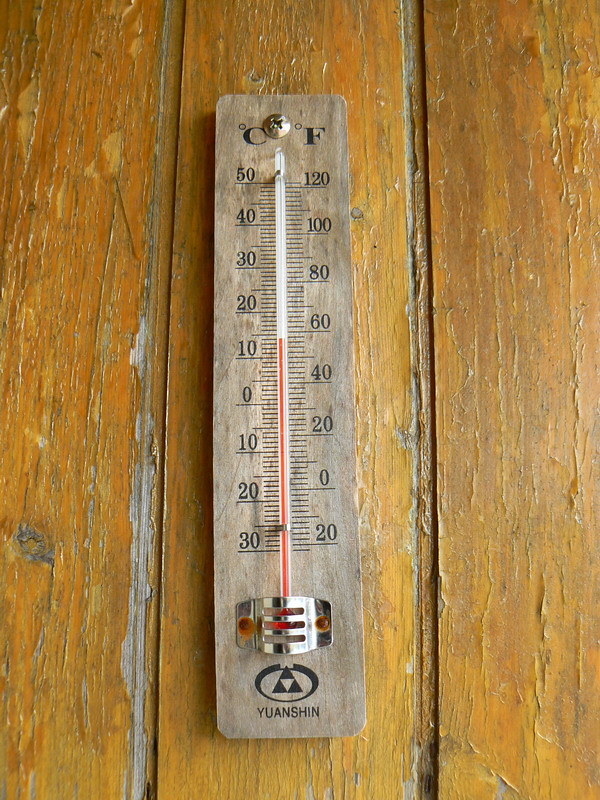The image showcases an old, rusted metal temperature gauge mounted on a weathered wooden wall composed of three distinct planks. The metal of the gauge is extensively corroded, except for the bottom holding mechanism and a screw, both of which appear relatively new. The bottom of the gauge bears the inscription "Wanching" alongside a small triangular symbol enclosed in a circle. The left side of the gauge reads in degrees Celsius, marked at intervals of 50, 40, 30, 20, 10, 0, and 10, 20, while the right side reads in degrees Fahrenheit, marked at intervals of 120, 100, 80, 60, 40, 20, 0, and 20. Additionally, finer gradations denote smaller temperature changes. The wooden planks behind the gauge were once painted, though the paint is now peeling and the wood shows considerable age. Despite the overall worn appearance, the glass covering the gauge remains clear and clean.